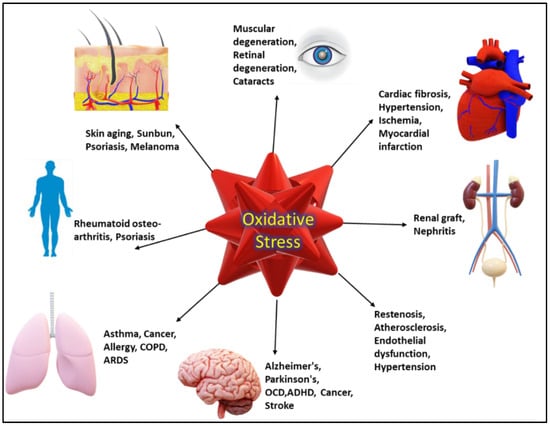The image appears to be an educational and medical diagram on oxidative stress, set against a white background. At the center is a red, symmetric geometric shape, reminiscent of an ornate wrapping paper bow, with yellow text outlined in blue that reads "oxidative stress." Surrounding this central shape are black arrows pointing outwards towards various organs and conditions, illustrating the widespread impact of oxidative stress on the body.

From the top, moving clockwise, the arrows point to:
1. Eye, accompanied by the conditions: muscular degeneration, retinal degeneration, cataracts.
2. Heart, linked to: cardiac fibrosis, hypertension, ischemia, myocardial infarction.
3. Kidneys, associated with: renal graft, nephritis.
4. Text describing vascular conditions: restenosis, atherosclerosis, endothelial dysfunction, hypertension.
5. Brain, detailing neurological conditions: Alzheimer's, Parkinson's, OCD, ADHD, cancer, stroke.
6. Lungs, indicating respiratory issues: asthma, cancer, allergy, COPD, ARDS.
7. Skin, showing dermatological effects: skin aging, sunburn, psoriasis, melanoma.
8. Overall human body, signifying general effects.

The diagram uses a color scheme consisting of red, gold, blue, white, pink, and purple, and includes diverse medical illustrations to visually represent the health issues affected by oxidative stress.